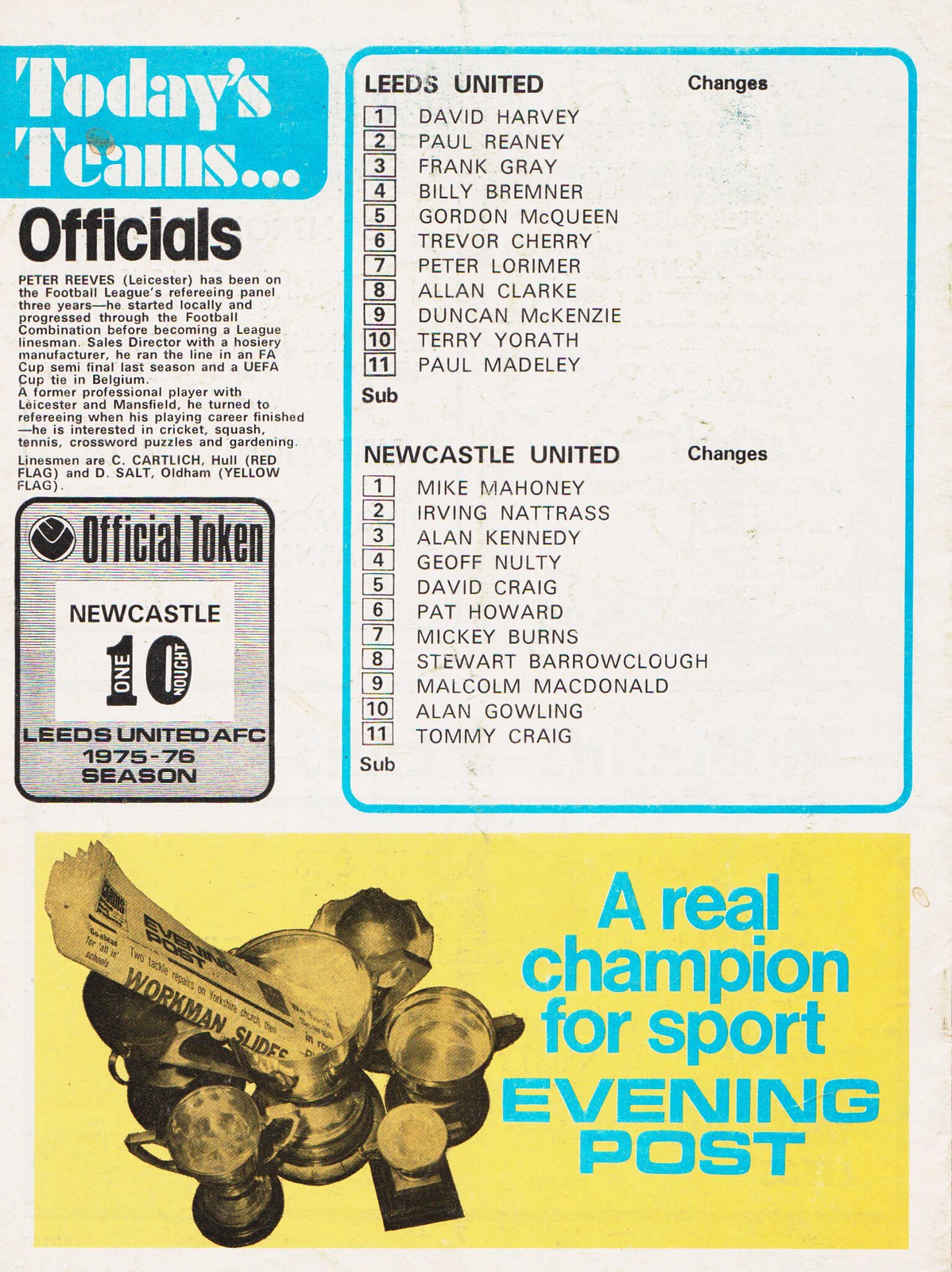This image features a vintage newspaper or magazine page with a slightly aged, grayed white background. The layout is compartmentalized into distinct sections with various details presented in bold and smaller print. In the top left corner, there is a light blue rectangle with beveled edges that reads "Today's Teams" in white print. Below this, in large bold black letters, it says "Officials," followed by detailed text about Peter Reeves, a Leicester-based official who has been on the Football League's refereeing panel for three years. Additional information notes his interests and career transition from a professional player to a referee. Linesmen C. Cartlidge of Hull (Red Flag) and D. Salt of Oldham (Yellow Flag) are also mentioned.

Further down, a black square with beveled edges marks the "Official Token" for Leeds United AFC, 1975-76 season. Inside this black square is a smaller white square containing "Newcastle 10," with a unique formatting where "1" is written as "one" and "0" as "nought." Adjacent to this is a blue-outlined rectangle that lists team changes for "Leeds United" and "Newcastle United," following the same format with player names numbered 1 to 11 for each team. For Leeds United, the players listed are David Harvey, Paul Harini, Frank Gray, Billy Bremner, Gordon McQueen, Trevor Cherry, Peter Lorimer, Alan Clark, Duncan McKenzie, Terry Yorath, and Paul Madley. Corresponding players for Newcastle United are Mike Mahoney, Irving Natras, Alan Kennedy, Jeff Nolte, David Craig, Pat Howard, Mickey Burns, Stuart Barrowclough, Malcolm McDonald, Alan Gowling, and Tommy Craig.

At the bottom of the page, there is an orange rectangle in landscape orientation. On the left within this rectangle, there is a grayscale image of several trophies with a newspaper placed in one. To the right, in light blue print, the text reads "A Real Champion for Sport, Evening Post."